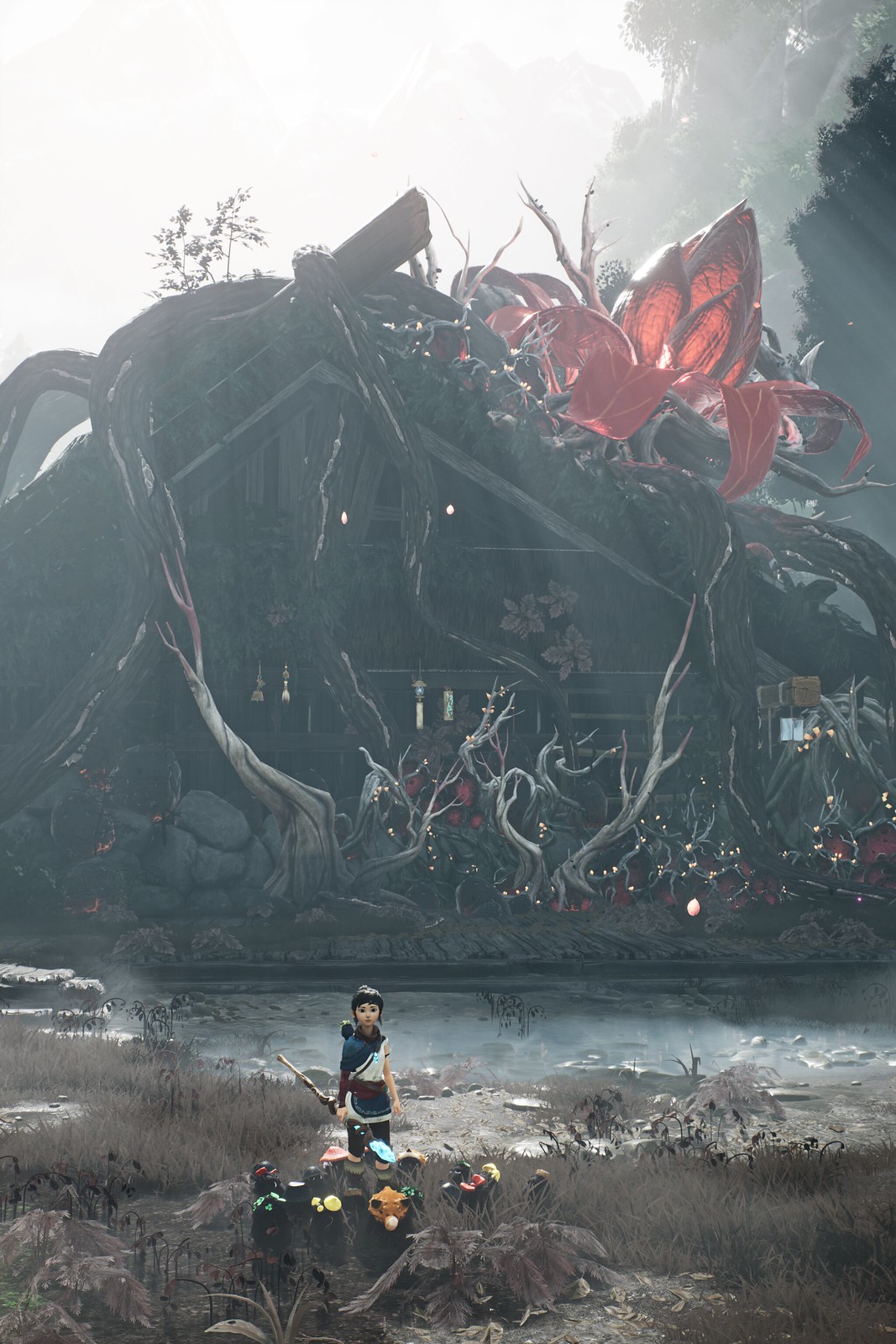In this detailed 3D video game screenshot, the main focus is on a character positioned slightly off-center to the left. This character is a young individual with long black hair, which is tied back—possibly in a bun or ponytail—and features short-cut bangs. They are dressed in a dark blue and white striped tunic that intriguingly combines asymmetrical elements: a long sleeve on the left arm while the right arm remains bare. Complementing this outfit are dark brown short pants and fur-like boots in shades of dark gray and brown.

In the background, there's an unusual, triangular-shaped house that seems integrated into the natural environment, likely built around an upturned tree's extensive root system. Adding to this unique setting is a large, glowing red flower emerging from the house's roof. The scene is illuminated by sunrays breaking through an overcast sky, creating a bright but diffused light. The backdrop includes a rocky structure that could be a distant mountain, dotted with dark-colored trees and various bushes, adding to the rugged, natural atmosphere.